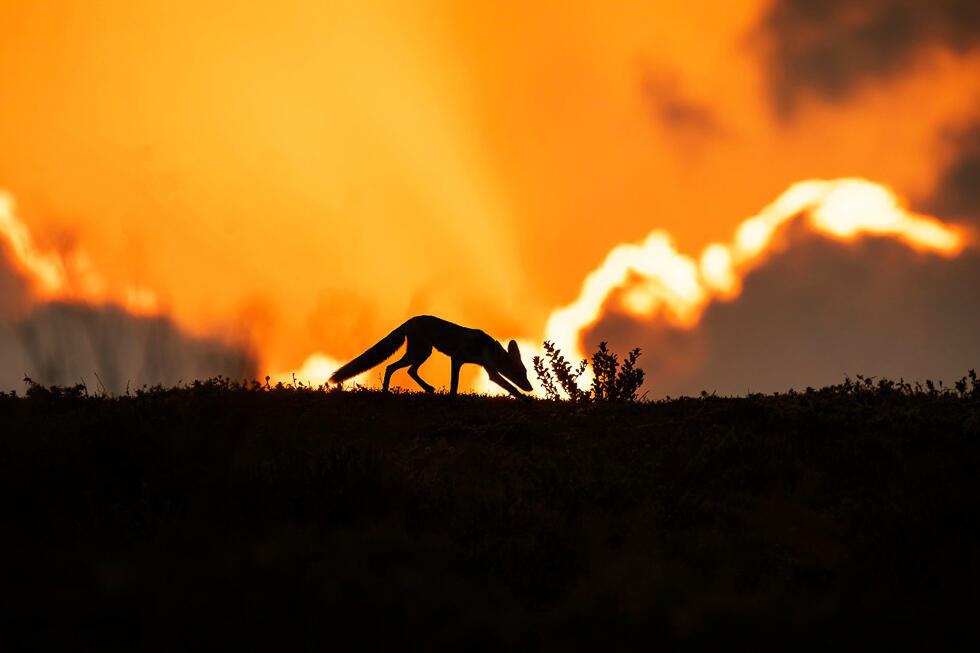The photograph features a dramatic sunset scene with a silhouetted animal, possibly a hyena, small wolf, or fox, walking on a steep hill. The sky is an intense orange with the tops of clouds visible to the right, creating a striking atmospheric backdrop. The foreground is completely dark, emphasizing the silhouette of the animal with its head lowered towards a bush or group of plants on the hilltop. The scene is accentuated by the outline of grass and weeds at the top of the hill. The animal’s tail is pointed downward, and the lower half of the image is entirely black, highlighting the stark contrast between the silhouetted foreground and the vivid sky. This artistic wildlife photograph captures the serene and haunting beauty of dusk with a focus on natural elements and the silhouette of the animal, making it a compelling visual piece rather than a scientific one.